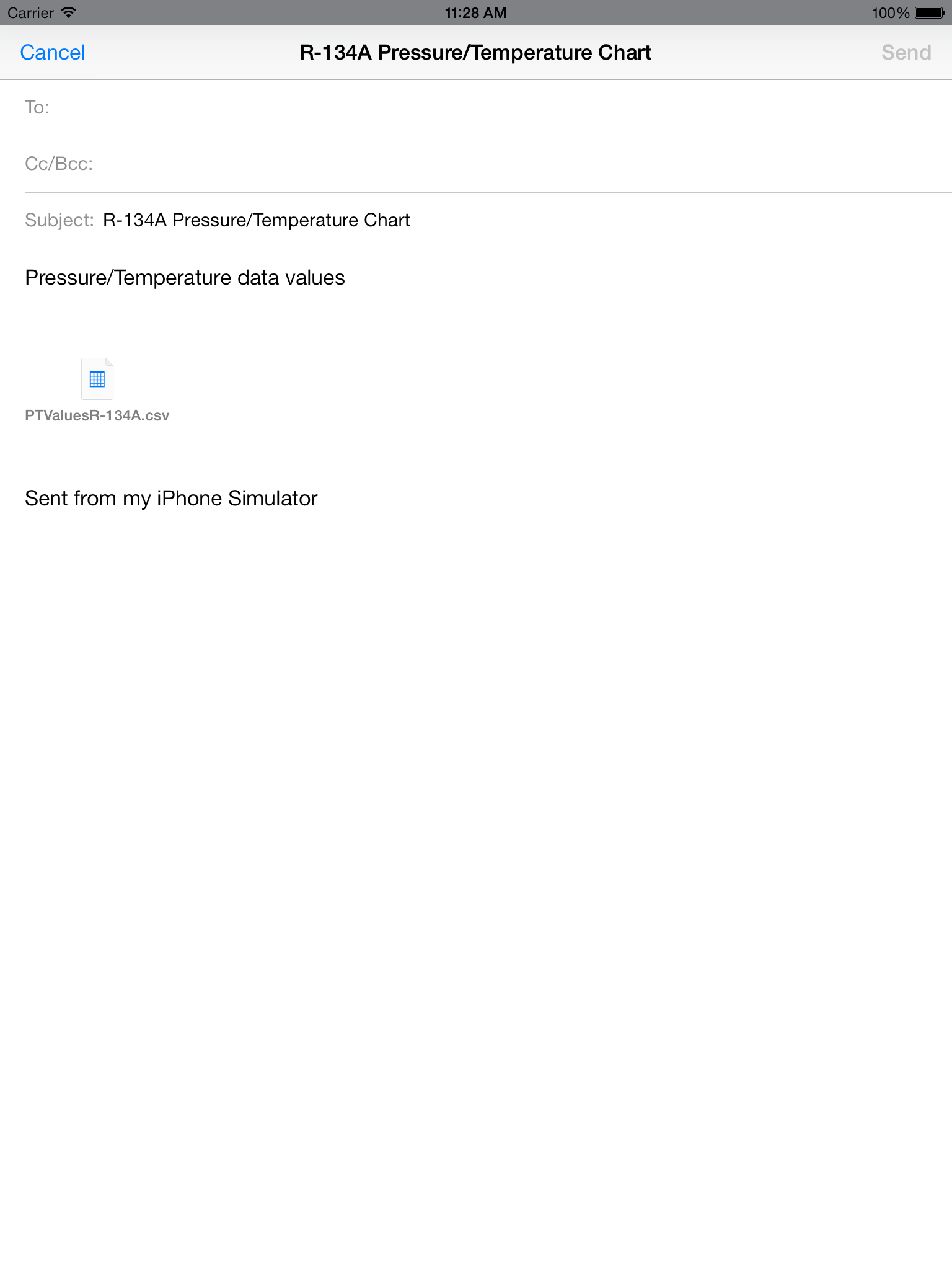This image appears to be a screenshot taken from a tablet or smartphone, as indicated by the black notification bar on the left-hand side. The notifications show the carrier name within a dark gray, slightly opaque rectangle, accompanied by a full wireless signal symbol. At the center of the notification bar, it displays the time "11:28 a.m.," whereas the far right side shows a fully charged battery icon. 

Central to the screenshot is a pop-up window framed by a light gray bezel. On the left-hand side of this window is blue, clickable text that says "Cancel." In the center, in black text, it reads "R-134a Pressure/Temperature Chart," with the initial letters "P," "T," and "C" capitalized. The right side contains the word "Send" in gray, with a capital "S."

Below this header, the interface resembles an email composition screen. The fields "To," "CC/BCC," and "Subject" are labeled in gray, with "T," "CC," and "BCC" capitalized. The "To" field has an ellipsis suggesting undisclosed recipients, while the "Subject" field contains the same "R-134a Pressure/Temperature Chart" title.

Within the email body, it details pressure/temperature data values, attaching a file icon that resembles a white sheet of paper with interconnected blue squares. The attached file is labeled in gray as "TP/TV Values R-134a.csv." Below the email body, in bold black text, it reads "Sent from my iPhone simulator."

This comprehensive caption paints a detailed picture of the screenshot, covering all visible elements in the interface.